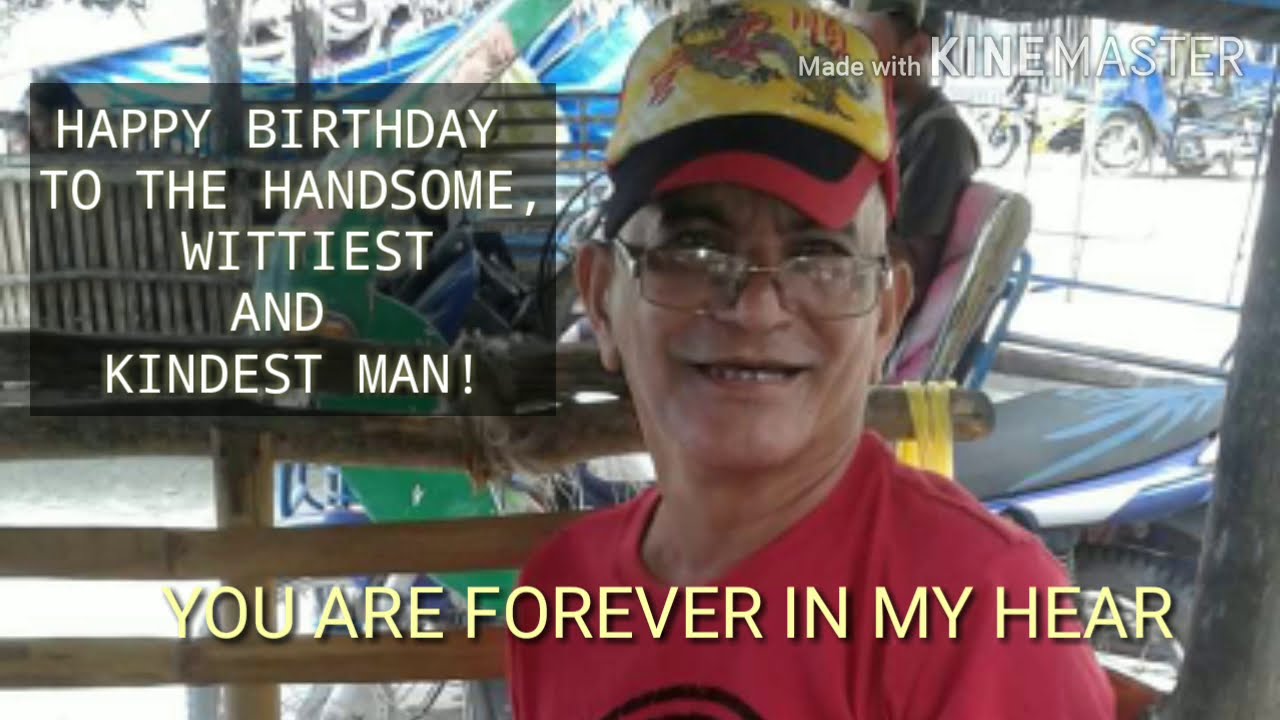In this vivid and celebratory image, we see an older man of around 55 years with light brown skin, smiling warmly at the camera. He sports a yellow, black, and red baseball hat adorned with a tiger design and wears glasses perched halfway down his nose. A bright red t-shirt completes his casual, cheerful look. Seated comfortably on a wooden bench, he appears to be in an outdoor storage area, possibly a backyard, with a variety of objects including piles of wood and plastic to his left, and parked motorcycles or bicycles in the distance to his right. A slatted wooden fence further frames the scene to the upper left.

Overlaying this snapshot of joy and nostalgia are heartfelt captions: in a shadowed box on the top left, it reads, "Happy Birthday to the handsome, wittiest, and kindest man!" At the bottom of the image, a slightly flawed yet touching message declares, "You are forever in my here," clearly meant to say "forever in my heart." This image, indicative of a screen capture from a personalized video made with the KineMaster app, encapsulates a moment of affection and celebration, immortalizing the man's birthday in a style reminiscent of a social media post.